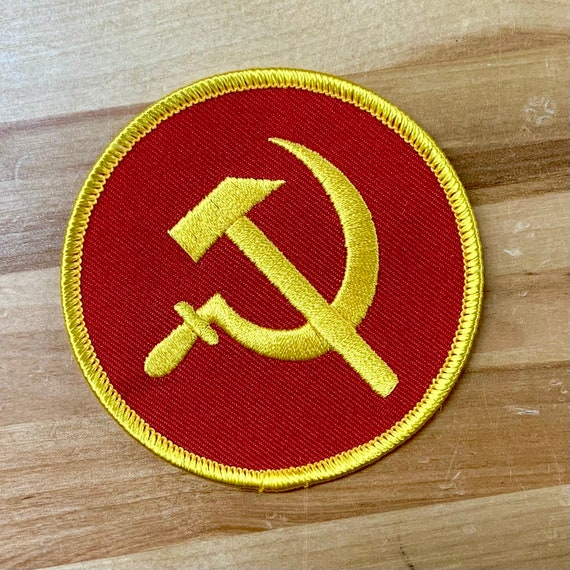This image features a round iron-on patch prominently placed on a wooden surface, likely a table. The patch boasts the iconic symbol of communism, the hammer and sickle, intricately embroidered in a yellowish-gold color. The background of the patch is a vivid red, enhancing its striking appearance. The hammer and sickle are crossed, with the sickle resembling a crescent moon with a handle and the hammer featuring a long handle with a head shaped somewhat like an axe. The yellowish-gold embroidery also outlines the patch, providing a neat, finished look. The wooden surface beneath the patch has a distinct wood grain texture, light in color with occasional darker spots, giving a rustic contrast to the vibrant patch. The image captures the patch lying flat, centered in the middle of the wooden backdrop, emphasizing its detailed craftsmanship and design.